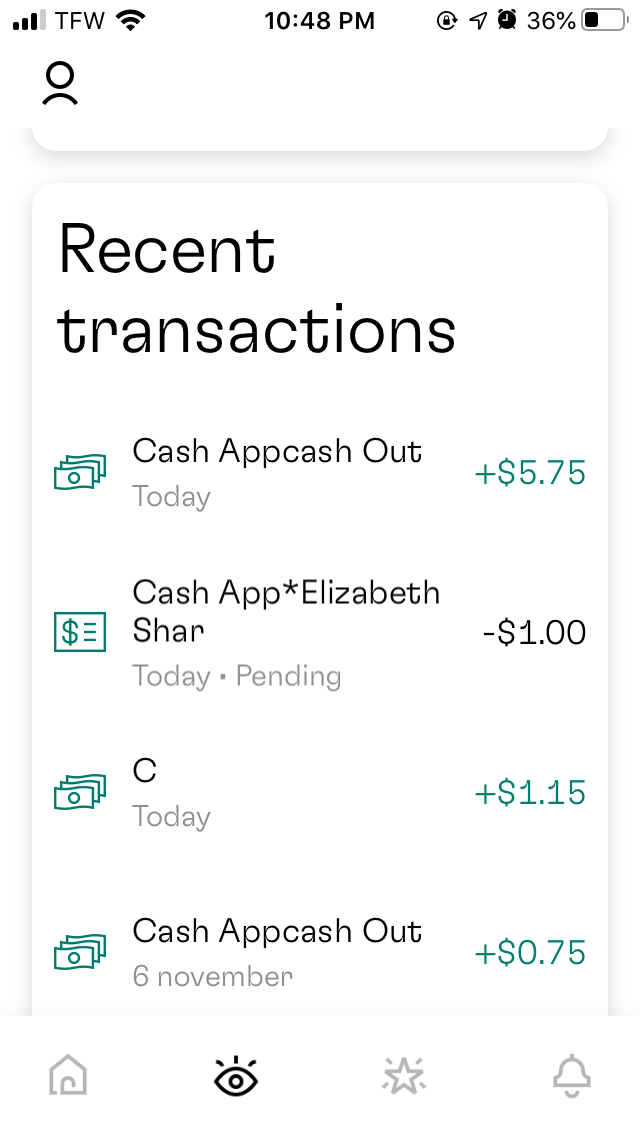This screenshot captures the interface of a financial application on a mobile phone, highlighting recent transactions. At the top, the section is titled "Recent Transactions." The first entry shows a "Cash App Cash Out" transaction from today, marked in green with a positive balance of $5.75, accompanied by an icon of some dollar bills. The second entry is labeled "Cash App *Elizabeth Shar" for today, currently pending, with a deduction of $1 in black text, illustrated with a dollar sign within a rectangular box. The third transaction displays "C," marked with a green plus $1.15 for today, also featuring the dollar bills icon. The final listed transaction is another "Cash App Cash Out" from November 6th, credited with 75 cents, indicated in green and paired with the same dollar bills icon. At the bottom of the screen, there are four icons representing different functions: a house icon, an eye icon, a star icon, and a bell icon.